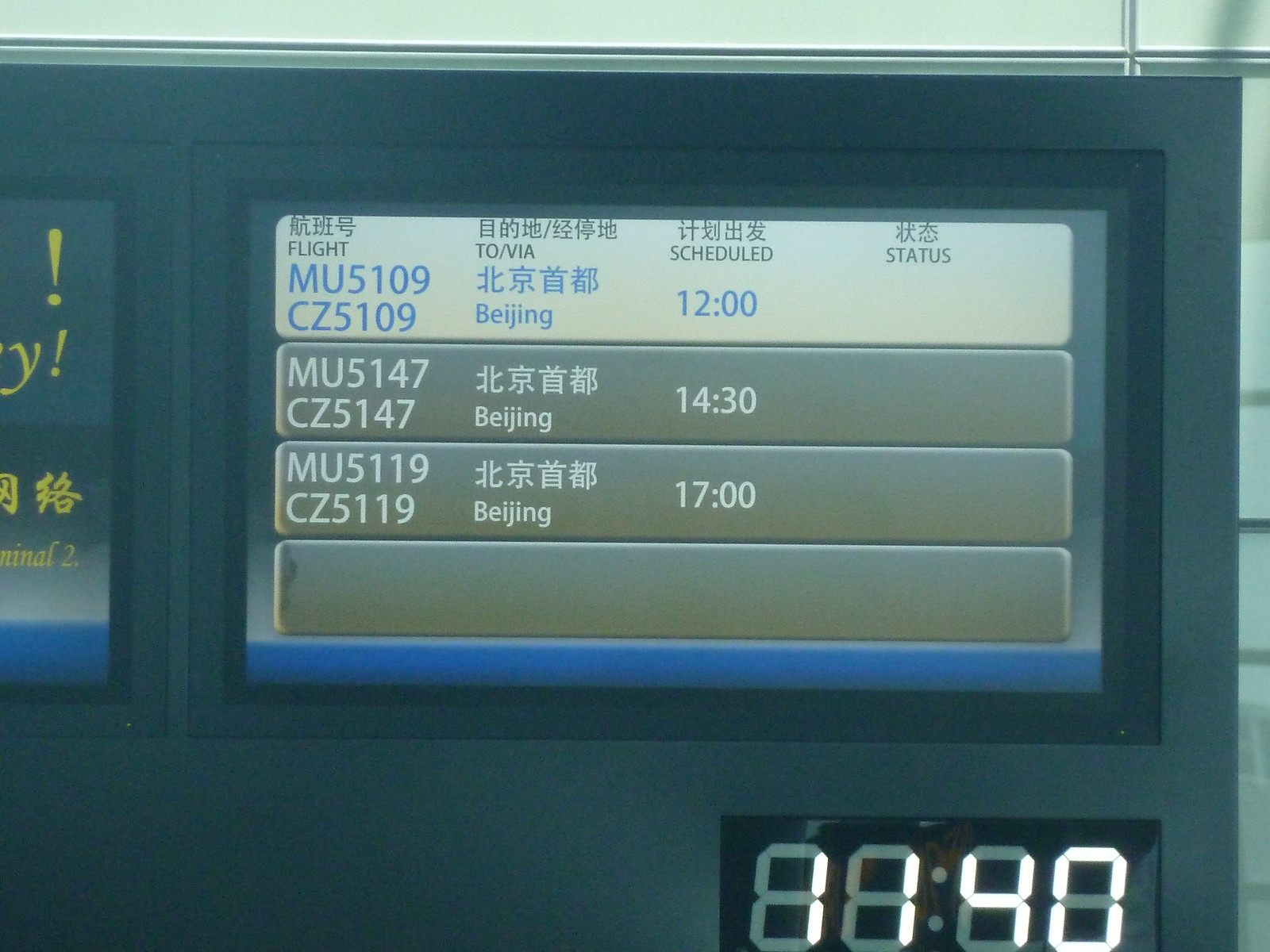This image is a close-up of a wide, rectangular flight status board found in an airport. The board, dark green with a silver border, features four rows of information, each displayed in a stacked light gray rectangle against a smaller, darker green rectangle. At the bottom, a digital clock shows the time as 11:40. The board lists flights MU5109 and CZ5109 to Beijing, scheduled for 12:00 with the status unspecified. The subsequent row lists flights MU5147 and CZ5147 to Beijing, scheduled for 14:30, followed by flights MU5119 and CZ5119 to Beijing, scheduled for 17:00. All text on the board is displayed in white, blue, and black, providing clear information on the upcoming departures to Beijing.